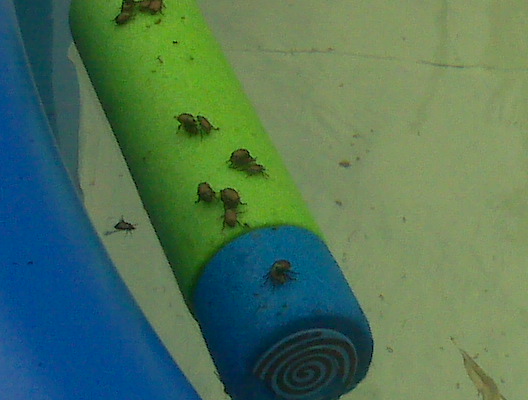The image features a detailed close-up of a green foam cylindrical object, likely found in a pool setting. The main body of the cylinder is green, while the end is a blue cylindrical piece adorned with an incomplete black swirl pattern. The background appears to be that of a pool, indicated by a floating brown leaf in the lower right and a blue circular plastic piece on the left, possibly the edge of the pool. Scattered across the foam cylinder are several small bugs that resemble oversized beetles or round six-legged insects, with appearances similar to small potatoes with legs. There is a notable concentration of bugs: four near the top, seven in the middle, and one on the blue end cap. Additionally, one bug appears to be floating lifelessly in the pool water.